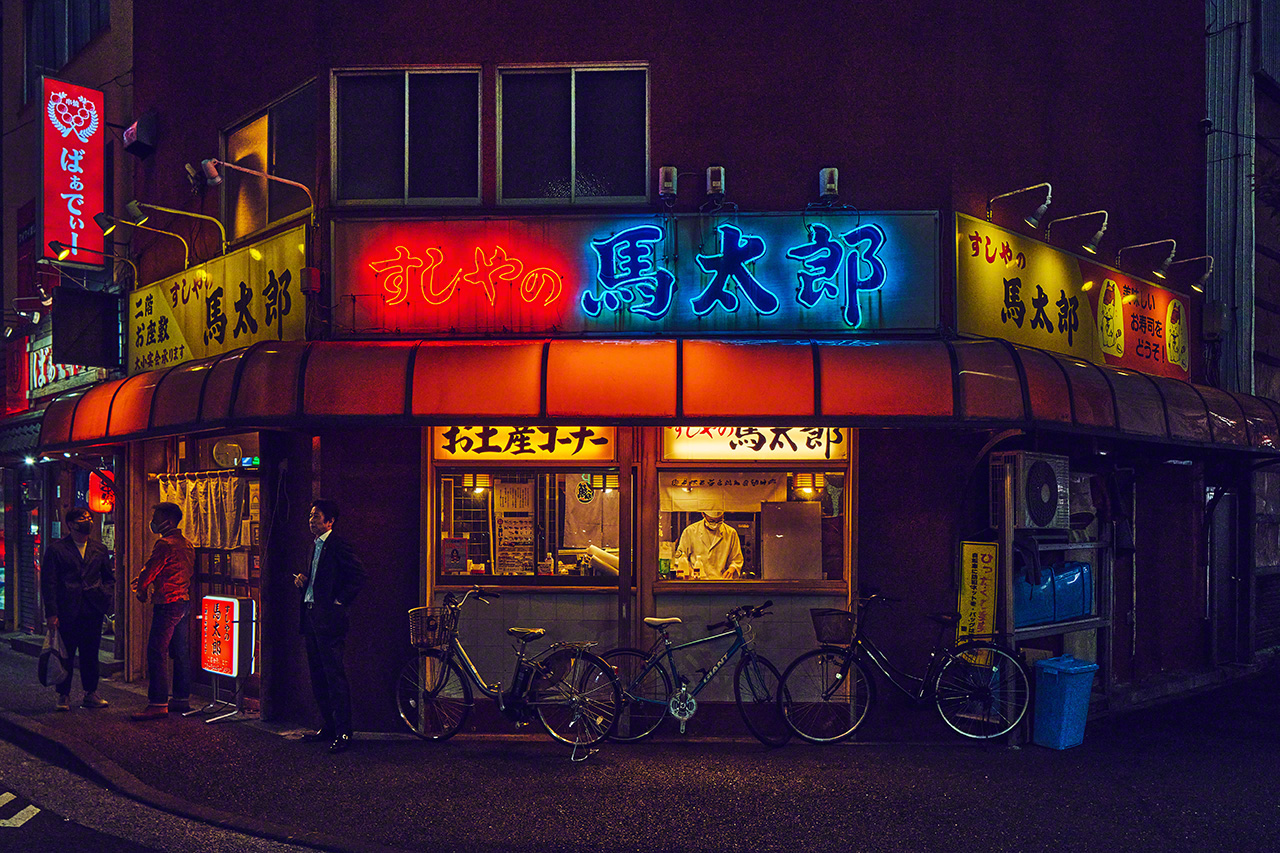This photograph captures a bustling street corner in Tokyo at night, showcasing a vibrant restaurant adorned with colorful neon signs in Japanese hiragana and kanji. The restaurant, located on a corner, features two large windows illuminated by warm yellow lighting from within, offering a glimpse of the interior where a masked chef, dressed in a white apron and headband, diligently prepares food in what appears to be a kitchen setting. In front of the windows, three bicycles are parked, suggesting patrons possibly arrived by bike. Nearby, three individuals stand casually; one in business attire appears to be smoking, while the other two, dressed in business casual outfits and wearing masks, engage in conversation. The exterior of the building also includes air conditioning units and trash bins. The scene is vividly marked by a red overhang that provides shelter from the rain, and a myriad of neon signs in red, blue, and yellow, which light up the establishment and add to the vibrant night-time ambiance of the city.